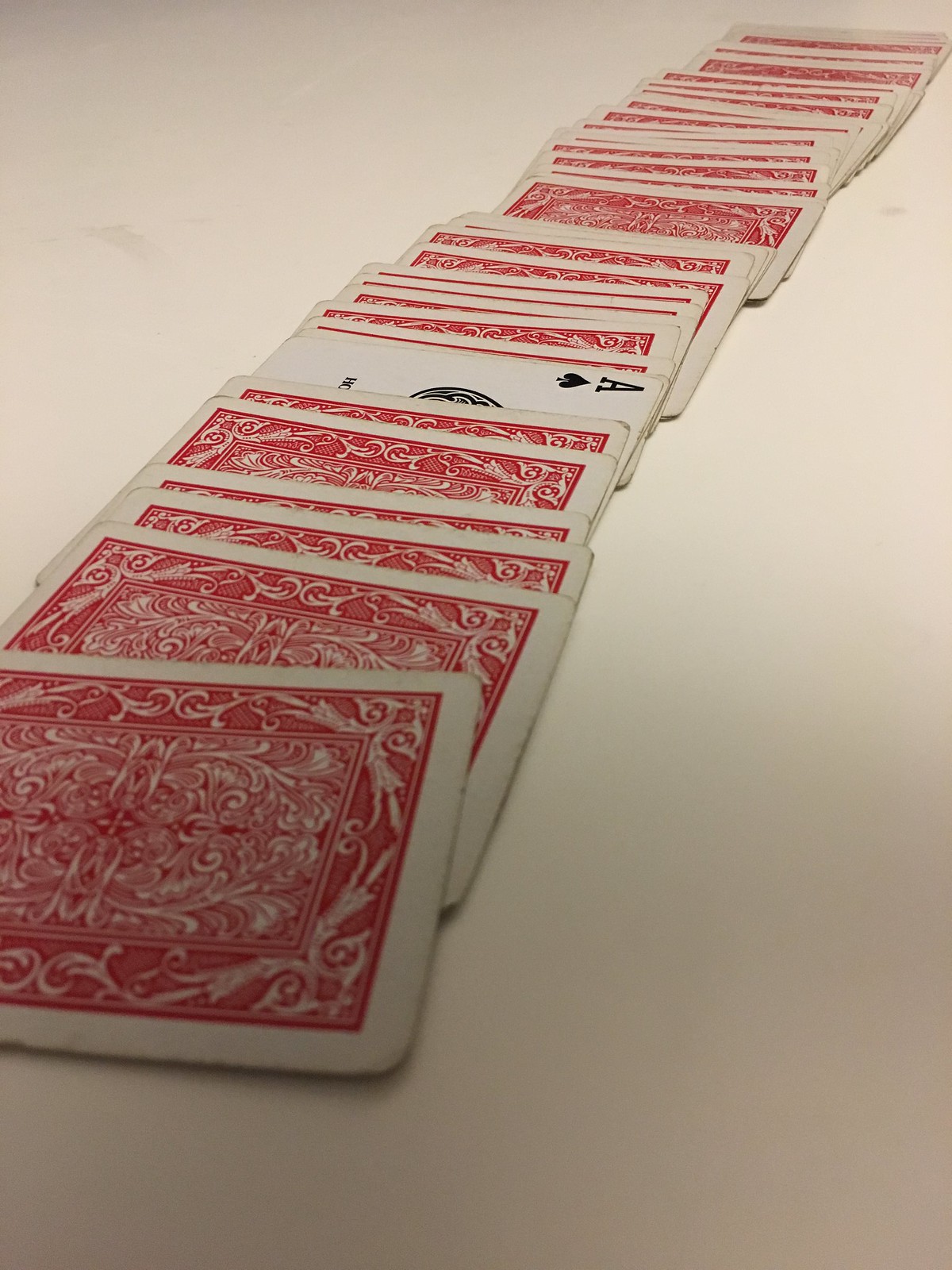A well-worn deck of cards is fanned out in a diagonal formation in this image, exhibiting clear signs of age and frequent use. The corners of the cards are noticeably worn and frayed, accentuating their vintage appearance. At the center of the spread, the ace of spades stands out, slightly lifted and prominently displayed, marked by yellowing indicative of time and handling. The cards are unevenly spaced, creating a slightly haphazard arrangement. They rest on a solid beige surface, the exact nature of which is indeterminate, possibly a floor or a table. Visible dirt marks sporadically adorn this surface, adding to the overall aged and weathered aesthetic of the scene. The backs of the cards feature a red pattern with white designs and a distinct white border encircling each one. While the total number of cards is unclear, the entire presentation evokes a sense of nostalgia and history.